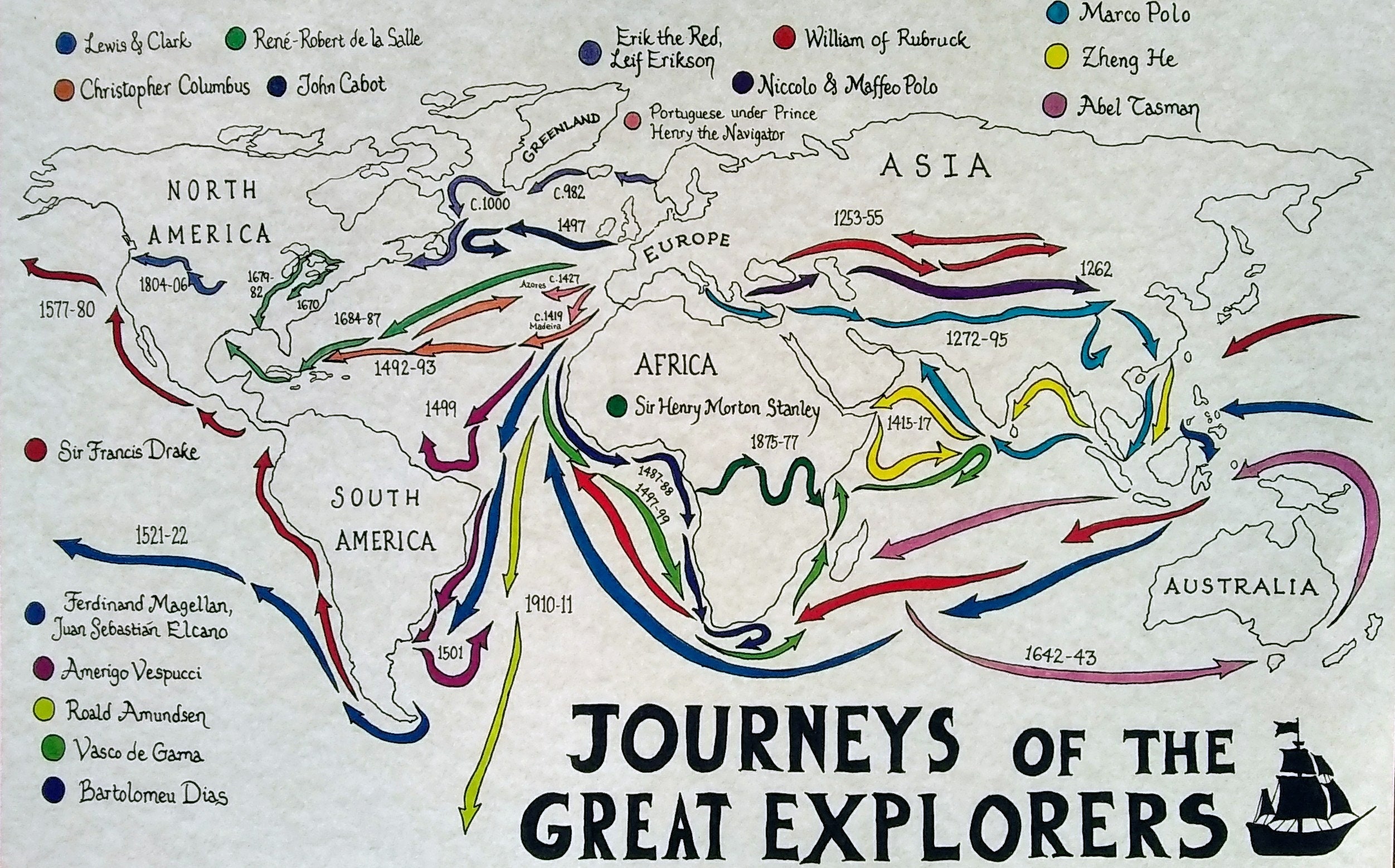This is an illustrated map titled "Journeys of the Great Explorers" in black text at the bottom, accompanied by an image of a Cutty Sark ship. The map features the continents—North America, South America, Europe, Asia, Africa, Australia, and Greenland—marked with various bright colored arrows and dates that trace the routes taken by multiple explorers. At the top, a legend with different colored circles matches each explorer to their respective routes: Lewis and Clark (blue), Christopher Columbus (orange), René-Robert De La Salle (green), John Cabot (black), Erik the Red (blue), Leif Erikson (blue), William of Rubruck (red), Niccolò and Maffeo Polo (black), Marco Polo (teal blue), Zhang He (yellow), Abel Tasman (pink), Sir Francis Drake (color not specified), Ferdinand Magellan (blue), Juan Sebastián Elcano (color not specified), Amerigo Vespucci (purple), Roald Amundsen (yellow), Vasco da Gama (green), and Bartolomeu Dias (dark blue). The detailed arrows depict the explorers' voyages, correlating with the dates of their explorations, making it both a visually engaging and informative map of historical journeys.